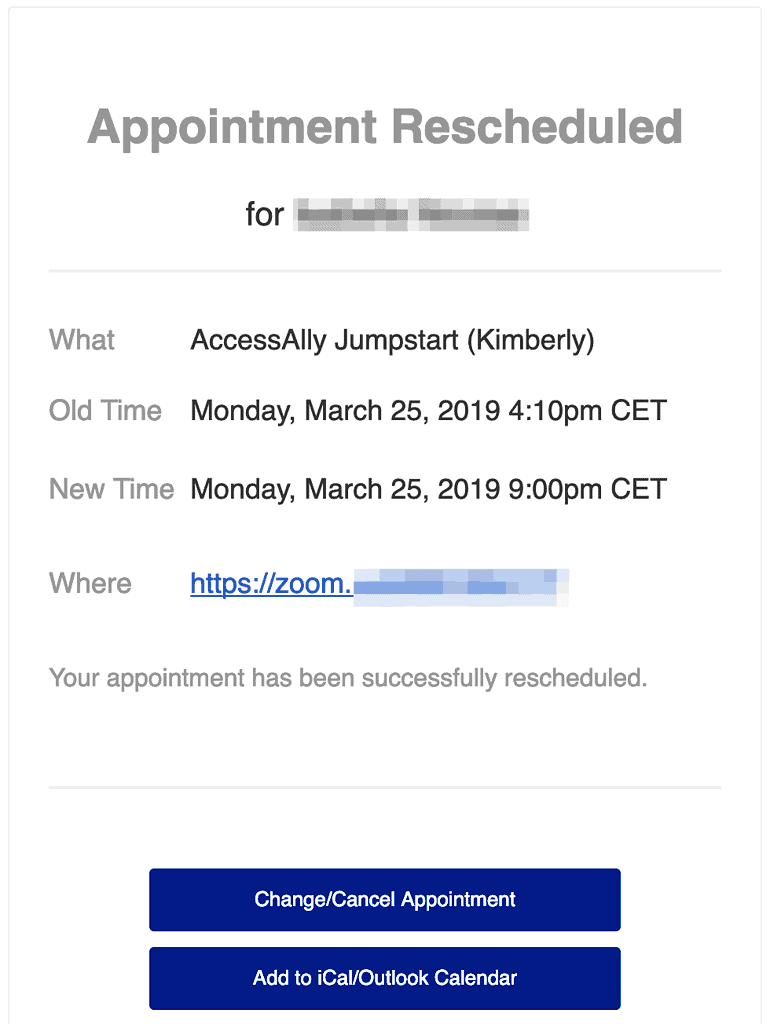The image appears to be an email notification about a rescheduled appointment. The notification is presented in a large white box outlined in faint gray. At the top section of the box, a horizontal line of text reads "Appointment Rescheduled For" followed by a redacted name. 

Below this is a faint gray line that separates the header from the details of the rescheduling. The text "Access Alley Jumpstart (Kimberly)" is displayed prominently. It specifies the old appointment time as "Monday, March 25th, 2019, 4:10 PM CET" and the new appointment time as "Monday, March 25th, 2019, 9:00 PM CET."

Further down, there is a section labeled "Where" with a hyperlink starting with "HTTPS://zoom." The rest of the URL is obscured. Following this, the text "Your appointment has been successfully rescheduled" is shown.

A second faint gray divider line appears, below which are two blue hyperlink buttons. The first button, labeled "Change/Cancel Appointment," is written in white text. The second button, also in white text, reads "Add to iCal/Outlook Calendar." Both buttons are clickable, offering options to modify or add the appointment details to a calendar.